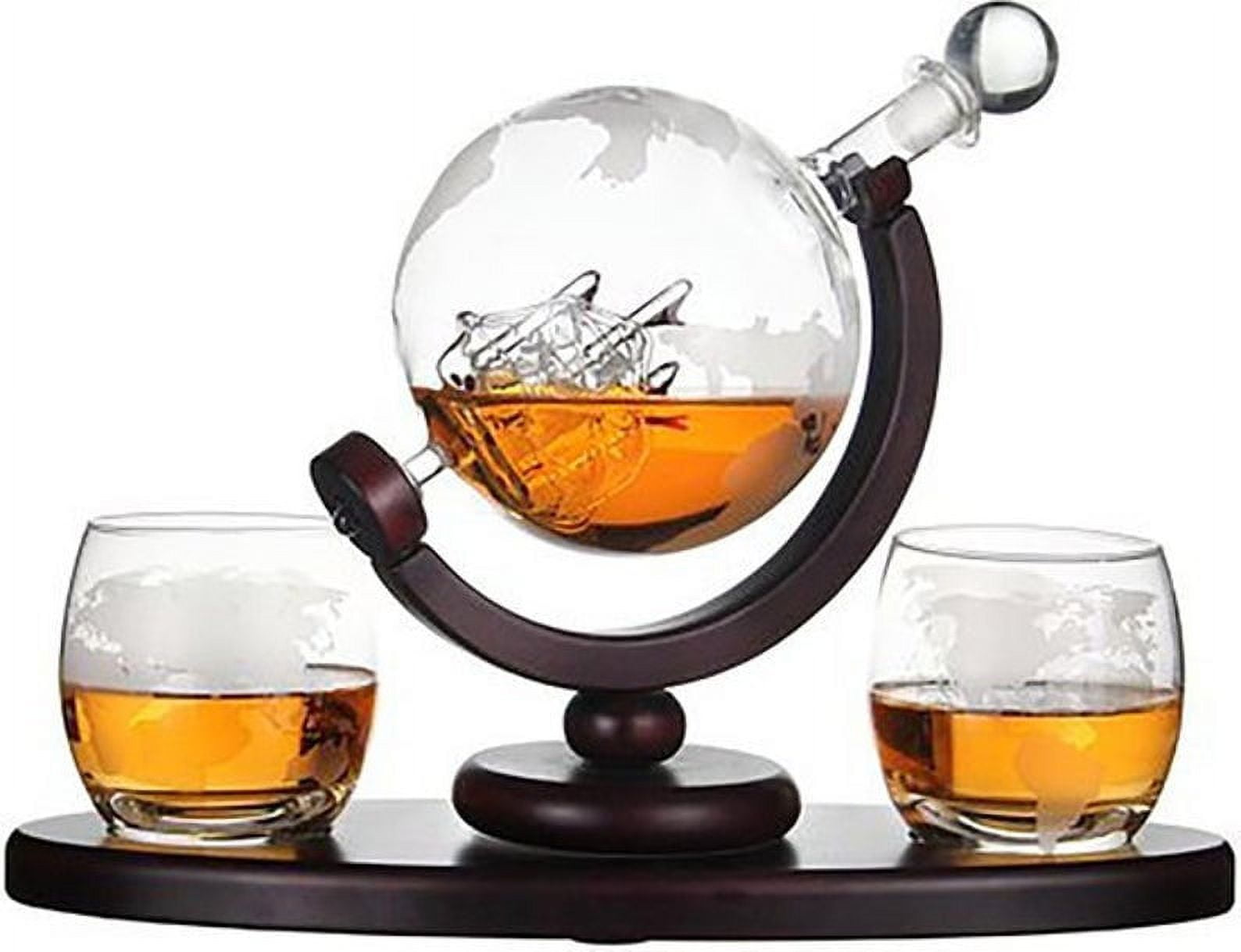This image depicts a unique and aesthetically pleasing whiskey serving set against a pristine white background. At the heart of the setup is a low-resolution photograph, but the elegance of the components is still discernible. The centerpiece is a round, crystal-clear glass carafe etched with a world map, containing a quarter-filled amber liquid, most likely whiskey. This globe-shaped carafe is tilted at a 45-degree angle and held in place by a custom-made, dark cherry wood stand. This stand includes a small circular base with a spinnable layer and an even smaller circle above that, ultimately connecting to a half-globe, C-shaped structure that cradles the carafe. On either side of the carafe are two matching clear glasses, each half-filled with the same amber liquid and featuring similar etched maps of continents. The entire arrangement, including the glasses and carafe, is set on a smooth, high-class wooden table, which adds to the luxurious aesthetic of the presentation.